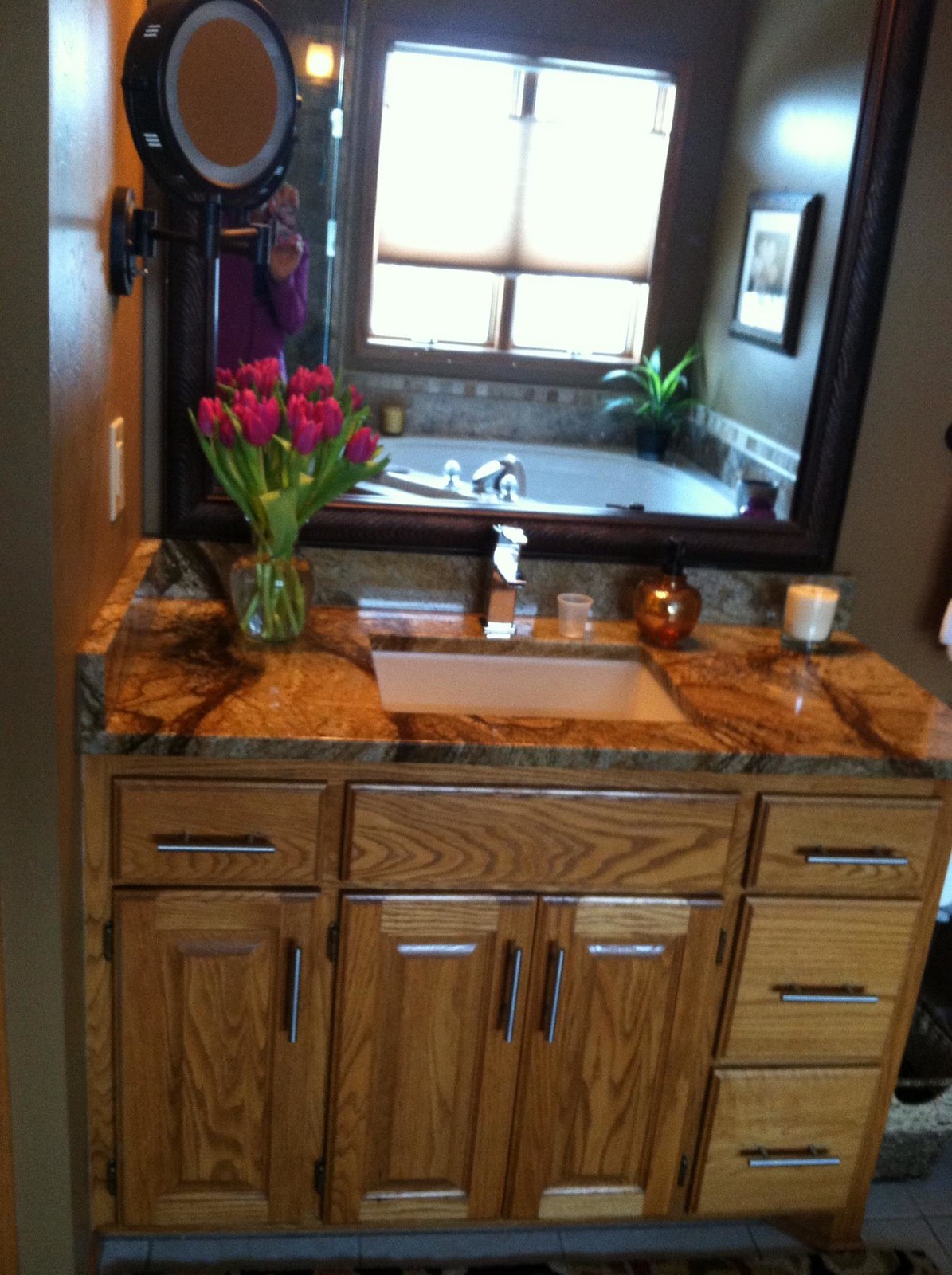The image captures an opulent bathroom, reminiscent of one found in a luxurious home. At the forefront, a sophisticated vanity area is in view, featuring a spacious countertop made of elegant marble or a similar high-end material. Positioned centrally is a pristine white sink.

The vanity's cabinetry, crafted from rich brown wood, consists of eight drawers, each adorned with sleek, gray metal handles. Notably, an upper drawer appears to have an unconventional pull-out design.

To the left on the countertop, a vase brimming with vibrant pink tulips adds a touch of natural beauty. To the right, a large white candle rests next to a brown hand soap dispenser and a small clear cup, providing both functionality and aesthetic balance.

Above the counter, a large black-framed mirror spans the wall, adding depth and dimension. Attached to the wall, in front of the mirror, is a smaller round magnifying mirror, likely used for detailed grooming tasks. The reflection in the main mirror reveals the photographer, distinguishably dressed in a purple shirt, with their face obscured by the magnifying mirror.

In the background, a spacious, round bathtub is visible, accentuated by a nearby green plant, which adds a hint of freshness to the serene scene. The tub is positioned under a large window, inviting an abundance of natural light and enhancing the overall air of tranquility and luxury apparent in this bathroom.